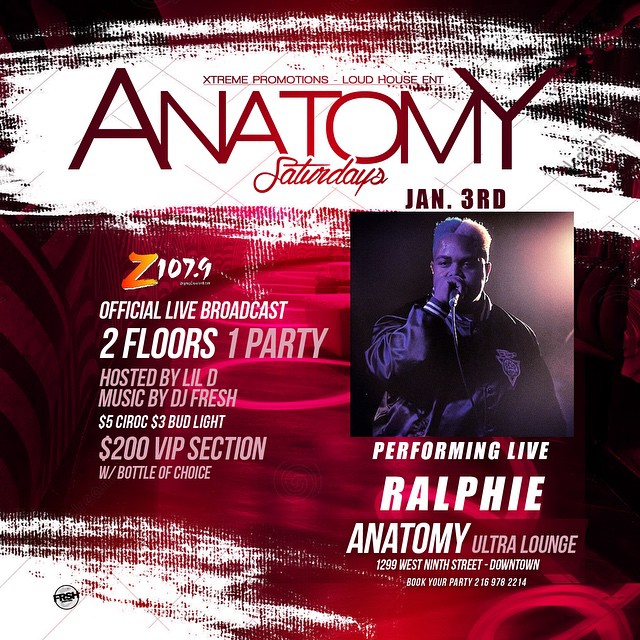The image is an advertisement for a live performance event at Anatomy Ultra Lounge. The background features a swirly mix of pink and red hues, with patches of black and a smeared white area at the center top. Prominently displayed in bold purple and red letters at the top is the word "Anatomy," with "Saturdays" written in cursive just below it. Underneath, the date "January 3rd" is noted. On the right-hand side, there's a photo of a dark-skinned individual wearing a satin baseball-style jacket, holding a wired microphone close to his mouth.

Above the photo, the date "Jan. 3rd, January 3rd" is repeated. Below, the text announces, "White Lettuce is performing live" followed by "Ralphie," spelled out R-A-L-P-H-I-E. Further down, additional details are provided: the event is at "Anatomy Ultra Lounge," with the address "1299 West 9th Street, Downtown." A promotional message invites attendees to "book your party," featuring a phone number, "216-978-2214."

Additional promotions on the left-hand side of the image include a live broadcast by radio station Z107.9 and the tagline "two floors, one party," hosted by Little D with music by DJ Fresh. Special offers are highlighted: "$5 Ciroc," "$3 Bud Light," and a "$200 VIP section" with a bottle of choice.

In summary, the detailed and vibrant advertisement captures the essence of the upcoming event, featuring live performances, exclusive offers, and enticing party details for January 3rd at Anatomy Ultra Lounge.